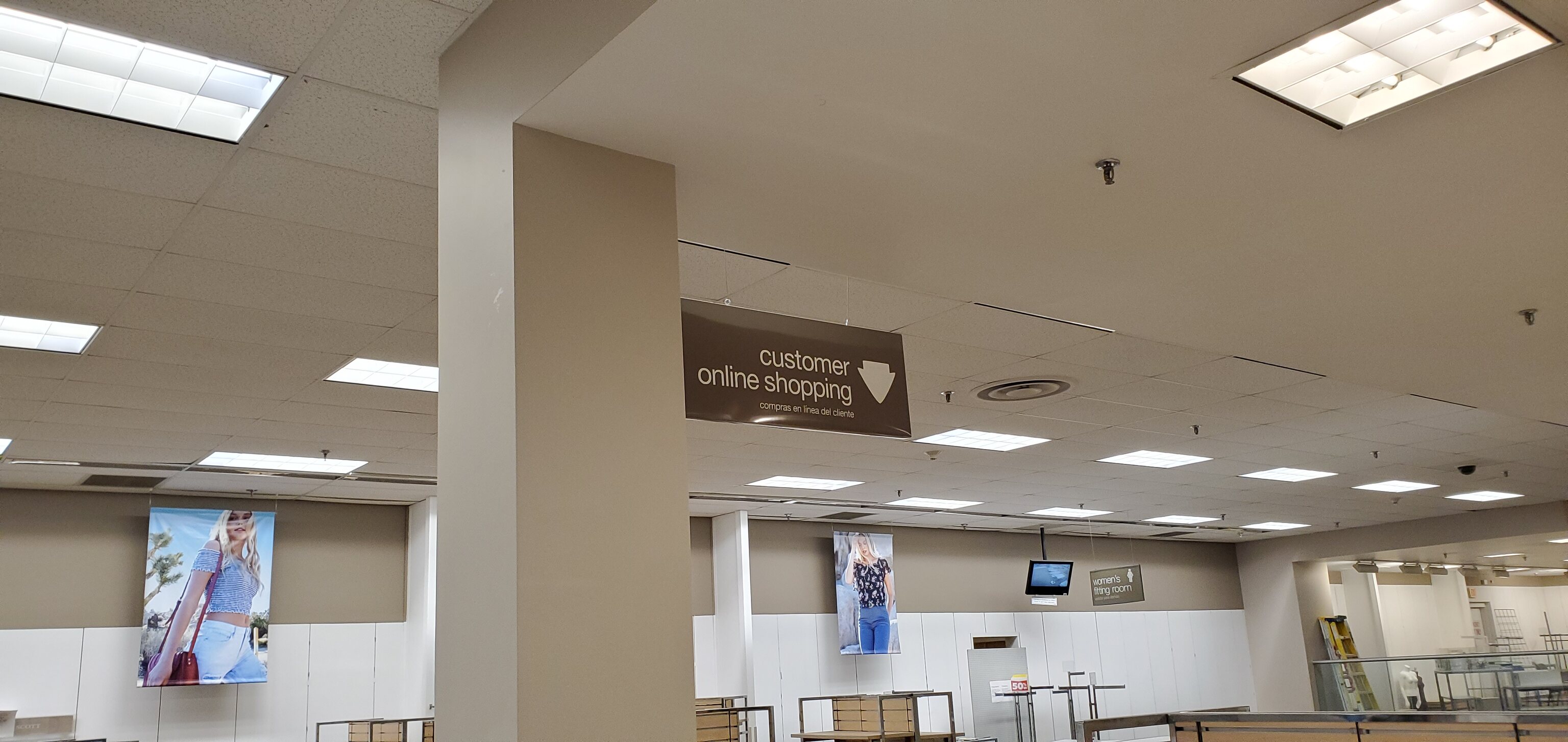The image depicts the interior of a seemingly empty retail store or a section under construction, possibly part of a shopping mall. Prominently featured on the bottom left is a large poster of a woman modeling an off-the-shoulder gray crop top, white jeans, and carrying a bag. Centrally located is a large tan pillar with a ladder propped against it. Above, a brown rectangular sign reading "Customer Online Shopping" with a downward white arrow hangs conspicuously. To the right, there’s another advertisement of a woman dressed in a black short-sleeved t-shirt with a print and blue jeans. The ceiling is fitted with fluorescent lights, industrial sprinkler systems, and other fixtures, with a TV mounted on one side. There are no visible products or shoppers; however, a few large push carts, tables, and chairs are scattered around, contributing to an overall feeling of incompleteness.